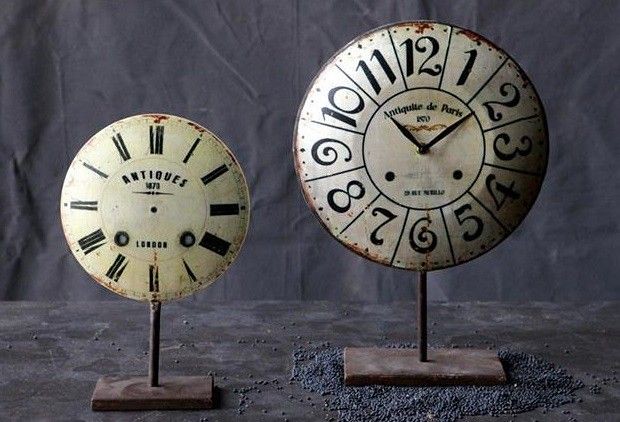This photograph captures two antique, weathered clock faces displayed on a metal stand, surrounded by a rustic, gravel-covered surface. The two clocks are mounted on slender metal rods that are anchored to a shared square metal plate. The larger clock, positioned on the right, is a faded whitish-beige with black Arabic numerals from one to twelve encircling its face. At the top, it reads "Antiquité de Paris," and the clock hands, both black, show a time of approximately 10:10, with the hour hand between ten and eleven, and the minute hand pointing at two. The smaller clock, on the left, features Roman numerals and has the inscription "Antiques" in its center, with a partially legible number below, and "London" above the Roman numeral for six. Both clocks exhibit signs of age, including rust and fading, and are presented against a backdrop of a grey, fabric-like curtain, enhancing the antique ambiance.